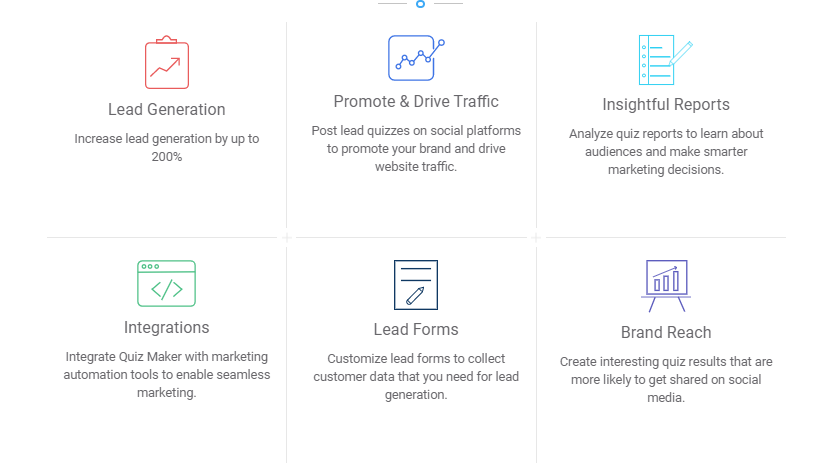In this infographic, two rows of three panels each present a series of marketing enhancement tools.

**Top Row:**
1. **Lead Generation**: A red box featuring an arrow pointing diagonally upwards symbolizes the potential to increase lead generation by up to 200%.
2. **Promote and Drive Traffic**: This panel emphasizes posting lead quizzes on social platforms to elevate brand promotion and boost website traffic.
3. **Insightful Reports**: Analyze quiz results to gather audience insights and make smarter marketing decisions.

**Bottom Row:**
1. **Integrations**: Seamlessly integrate QuizMaker with various marketing automation tools for streamlined marketing efforts.
2. **Lead Forms**: Customize lead forms to collect essential customer data required for effective lead generation.
3. **Brand Reach**: Craft engaging quiz results that are more likely to be shared on social media, expanding brand awareness.

The overall infographic is cleanly designed and employs eye-catching icons and images to effectively convey its message.